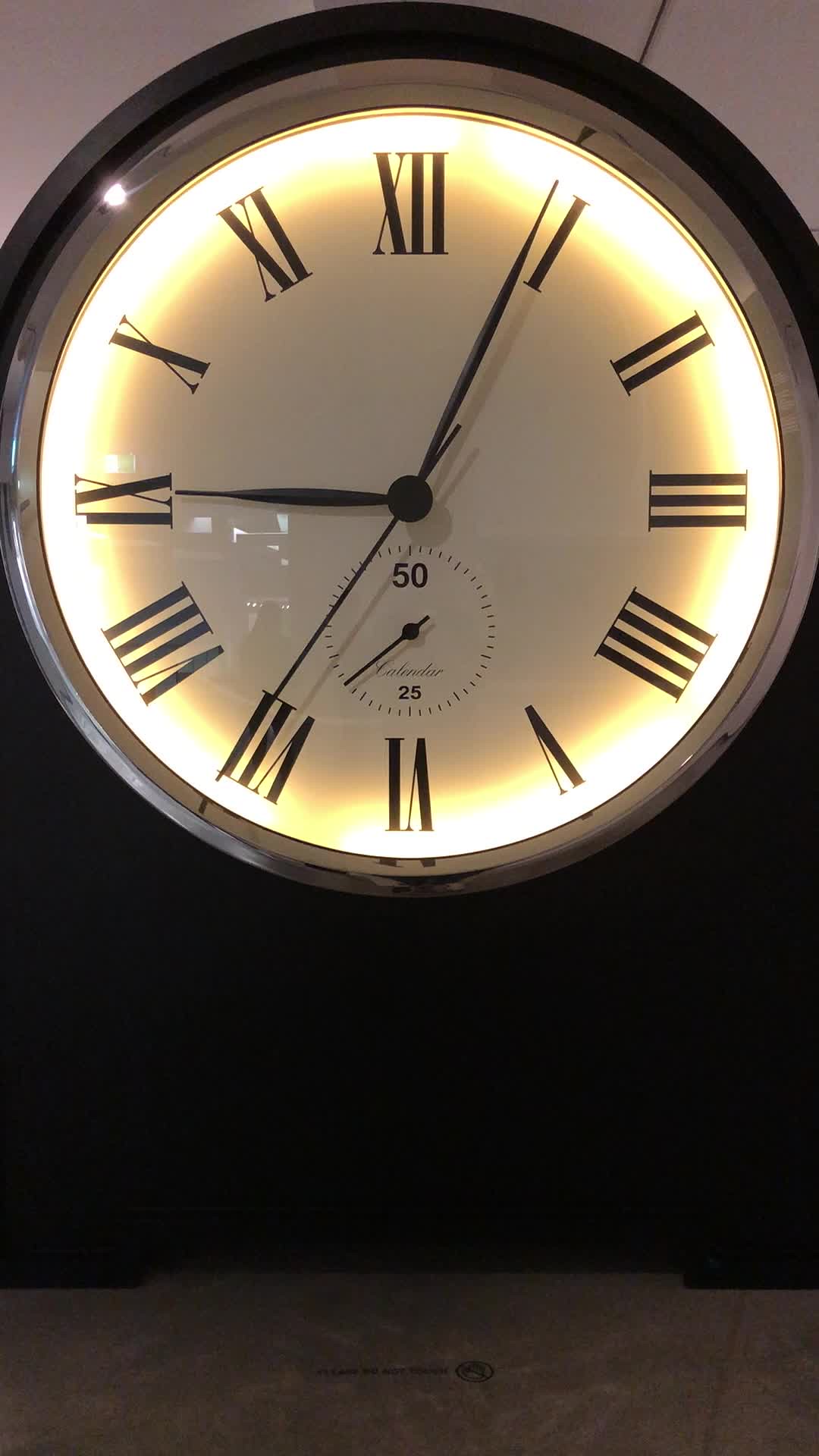The image features an elegant, circular mantelpiece clock, supported by a square, flat base with two small stubby feet positioned at the corners. The clock rests on a grey surface, exuding an air of classic sophistication. Its white dial is adorned with black Roman numerals, complemented by black hour, minute, and second hands. Beneath the main dial, a smaller sub-dial is prominently displayed, numbered 0 to 50 at the top and 25 at the bottom; its purpose remains unclear given the usual 60 seconds in a minute, adding a touch of intrigue to the design. Intricate wording lies beneath the sub-dial, though it is too small to decipher. The background is composed of white tiled surfaces, enhancing the clock's timeless appeal and suggesting it could seamlessly grace any mantelpiece with its presence.